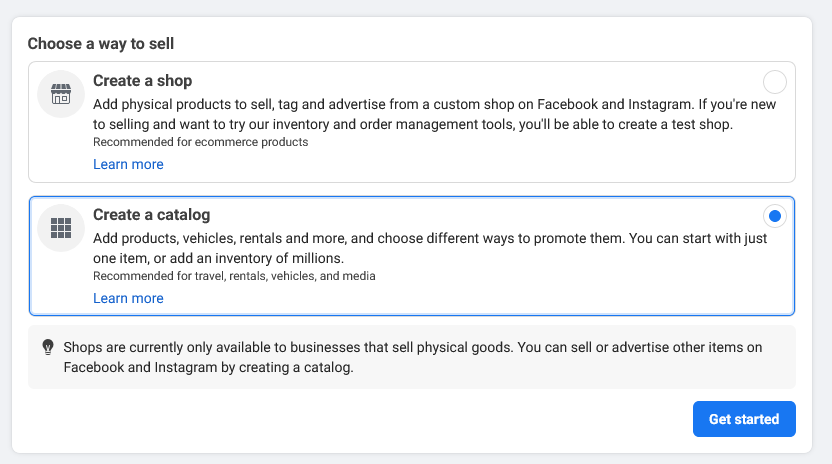In this image, we see a screenshot embedded within a light gray border. The screenshot features a white rectangular interface with options for setting up a selling platform. In the upper left corner, bold black text reads, "Choose a way to sell."

Below this heading, there are two white boxes presenting distinct options. The first box is outlined in gray and includes an icon of a house within a circular button. To the right of the icon, bold black text states, "Create a shop." Beneath it, smaller black text elaborates, "Add physical products to sell, tag, and advertise from a custom shop on Facebook and Instagram. If you're new to selling and want to try our inventory and order management tools, you'll be able to create a test shop."

The second box, highlighted in blue with a blue circle in the upper right corner, displays bold black text that says, "Create a catalog." The accompanying smaller text explains, "Add products, vehicles, rentals, and more, and choose different ways to promote them. You can start with just one item or add an inventory of millions."

At the bottom right corner of the screenshot, there is a blue action button labeled, "Get Started."